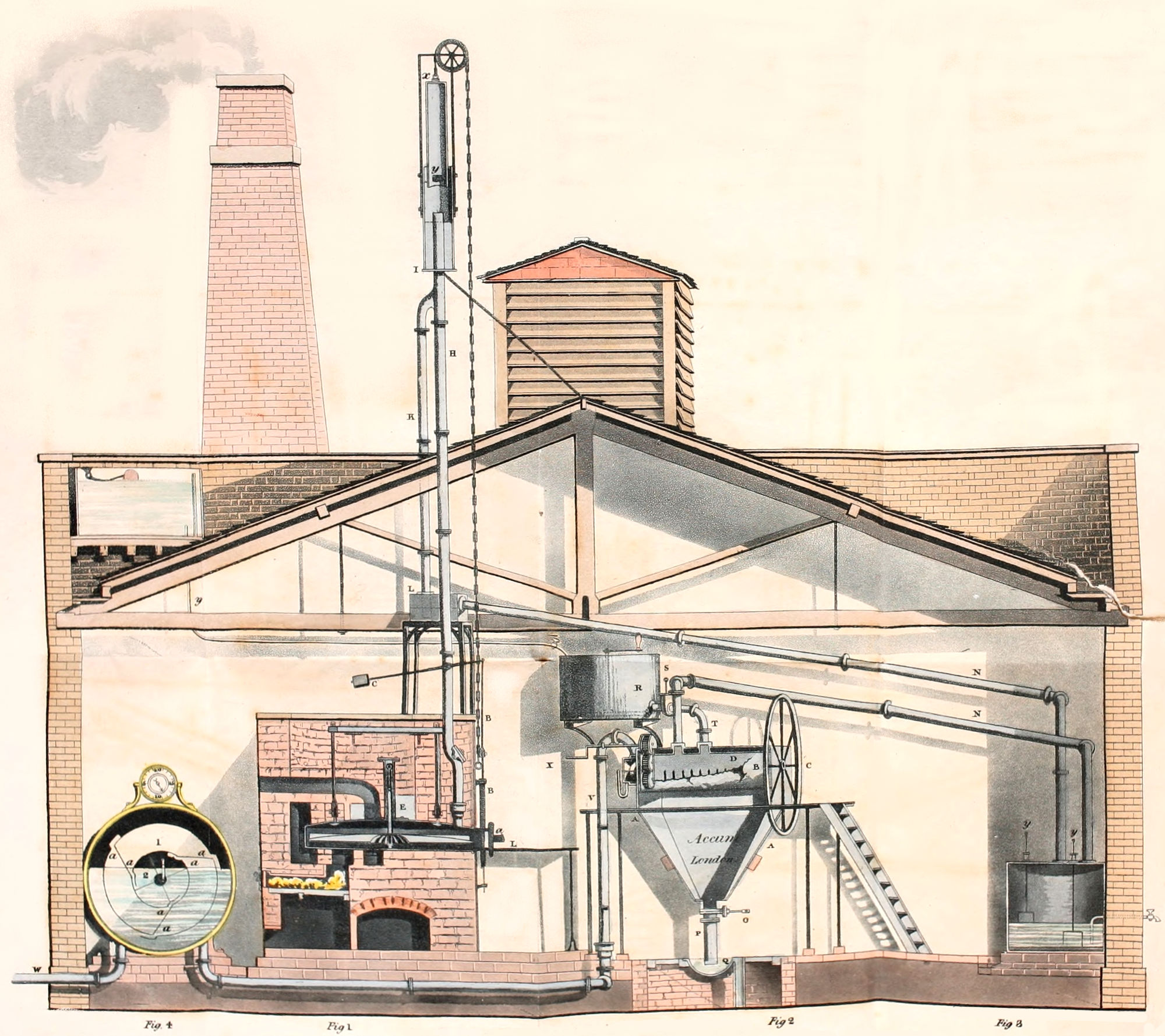This is a detailed, hand-drawn illustration of the interior of a brick building, presented as if the building has been halved to reveal its inner workings. The entire drawing is rendered in shades of pale yellow, reddish-pink, black, gray, and white, giving it an old-fashioned, almost antiquated look. A prominent chimney, located on the left side of the building, emits gray smoke into the air. Inside, a visible staircase leads to the center of the structure, where a large metal apparatus with a spinning handle is situated. This centerpiece is likely used for industrial purposes, possibly for sorting or processing materials such as seeds.

Throughout the building, interconnected pipes and tubes weave between various components, linking a fireplace made of brick to multiple other mechanical parts, including a silo. An A-frame roof support is visible, along with a smaller section of the building featuring wooden slats and a slanted roof. Near the bottom left of the image, there's a round device resembling a timer or monitor, containing water and connected to pipes. The comprehensive layout displays other elements such as funnels, sorters, and a metal pulley system that extends through the roof, emphasizing the scale and complexity of the machinery.

Additional details include small, annotated figures labeled “Figure 9”, “Figure A”, “Figure 2”, and “Figure 1,” though their specific references are unclear. The entire scene captures the essence of an industrial workspace, meticulously illustrated to showcase every intricate detail, set against a background of light coral pinkish hues.